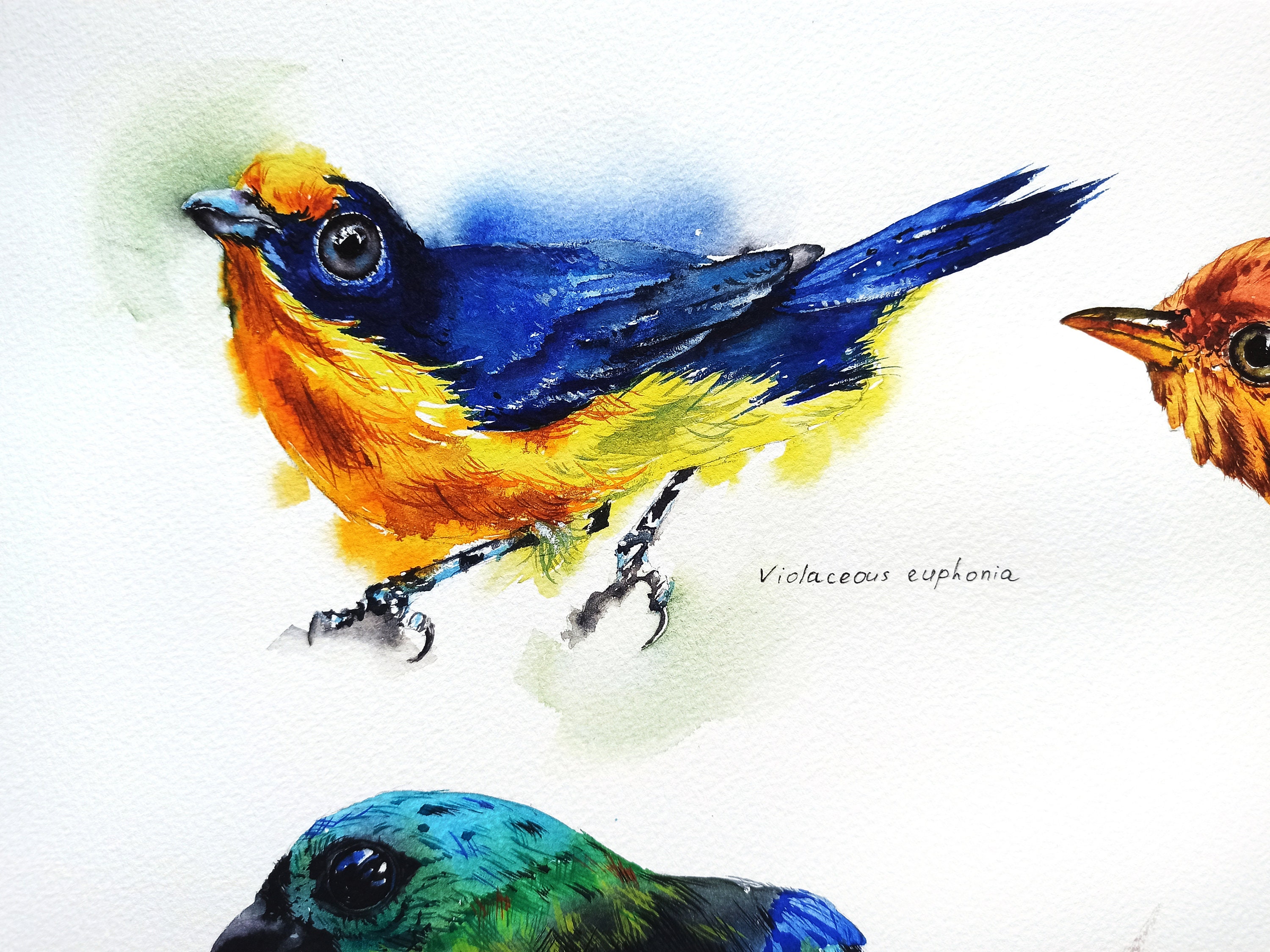The image features vibrant paintings of birds, with the focus on a fully-visible, small bird labeled as "Viola ceas euphonia." This main bird is strikingly colorful, with blue feathers on top, a yellow and orange belly, and bluish-gray legs. Its notable blue round eyes and a tuft of yellow feathers above its blue beak add to its vivid appearance. To the right, there is a cropped painting showing the orange face and beak of another bird, revealing just enough detail to see its eye. At the bottom, another partial bird appears, painted in shades of blue and green, with only its eye and some feathers visible. The white background of the canvas contrasts with the colorful birds, and there are some words in the image, including "euphonia" and a term that seems to read "violaceous." The paintings collectively showcase the vibrant and varied hues of these birds, emphasizing their beauty and intricate details.